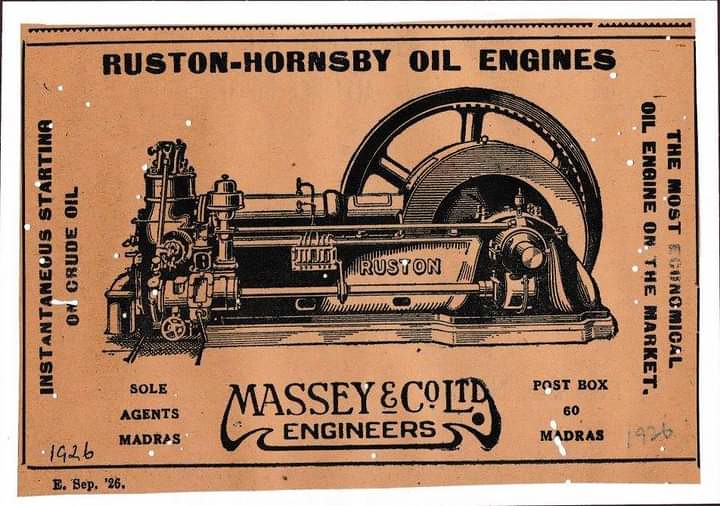The image showcases a highly detailed, zoomed-in view of a vintage advertisement or postcard, predominantly featuring an intricate black illustration of an engine labeled "Rustin" in the center. The background is a light brown color with white speckles, creating an aged, rustic appearance. At the top, the text reads "Rustin Hornsby Oil Engines" in bold black print. The advertisement touts the engine's capabilities, stating "Instantaneous starting on crude oil" and claiming it to be "The most economical oil engine on the market" with some faded and hard-to-read sections, such as "Massey and Colt engineers" adorned with an elaborate border at the bottom. The image predominantly comprises shades of white, black, brown, and hints of gray, effectively capturing the historic and industrial essence of the era.